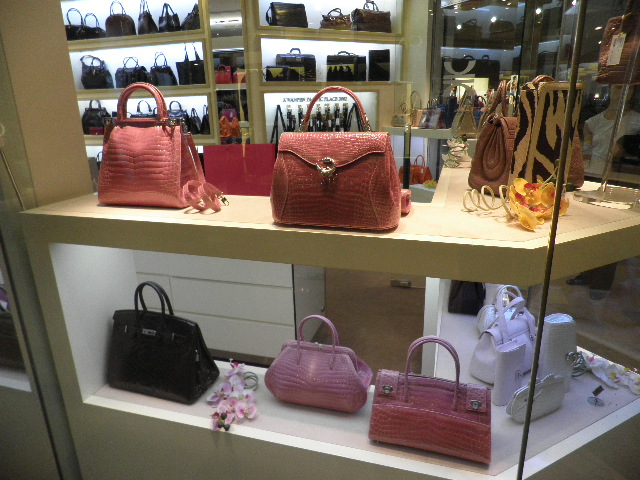The photograph captures an elegant store display showcasing various designer handbags. Positioned behind a glass cabinet, these purses rest on white and cream-colored shelves illuminated by specialized lighting that highlights their subtle sophistication. In the foreground, a collection of predominantly pink handbags in different shades stands out, accompanied by a sleek black bag, several white ones, and a tan-patterned purse. The upper shelf features another arrangement of pink handbags, including a particularly vibrant pink one, alongside a large brown-shaded bag and a selection of striped and dark brown handbags. The background reveals additional glass shelving filled with more handbags, suggesting that the store specializes in luxury purses made with cloth or leather handles. Each shelf on the back wall holds groups of four to eight purses, creating a visually appealing and well-organized display.